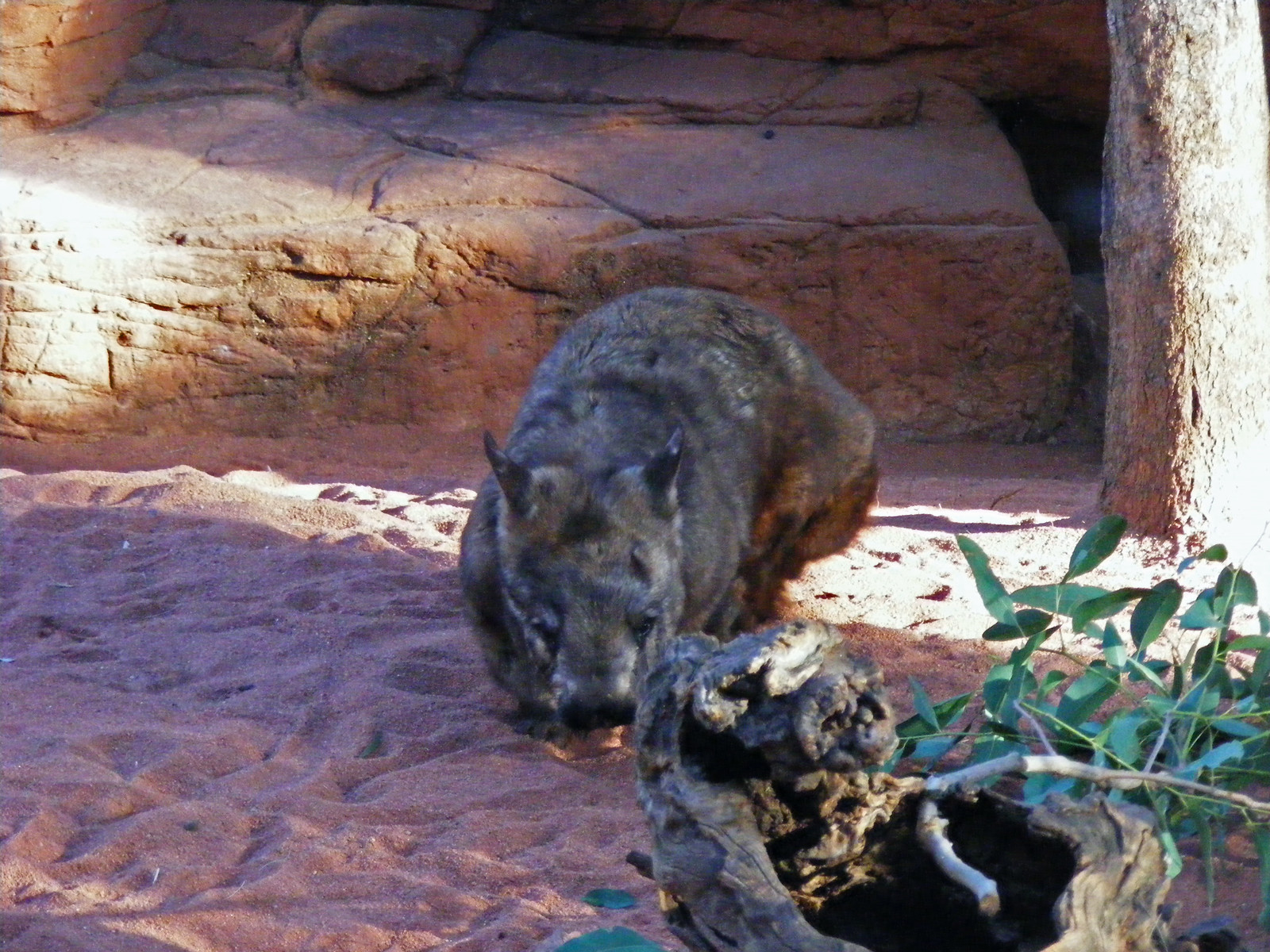In the center of this wide rectangular photo taken at a zoo, a small, furry, blackish-brown animal is sitting on a pile of reddish sand that fades to a yellowish hue on the right side due to light reflection. Its fur appears to have hints of greenish tones, possibly from the surrounding environment. The animal is positioned in a crouched, almost pouncing stance with its front paws beneath its head and its back right leg bent. It has sharp, upright black ears and a notable large snout, suggesting it might resemble a wolf or a feline, although its exact species is uncertain. The creature seems to be sniffing the ground. Near its right side, there's a large bushy tail visible. In the bottom right corner of the image, there's a gnarled wooden object with a branch attached, covered in thin green leaves that resemble eucalyptus. Behind the animal, there's an elevated structure made of reddish-gray, sandstone-like rocks, enhancing the zoo's rocky enclosure ambiance.